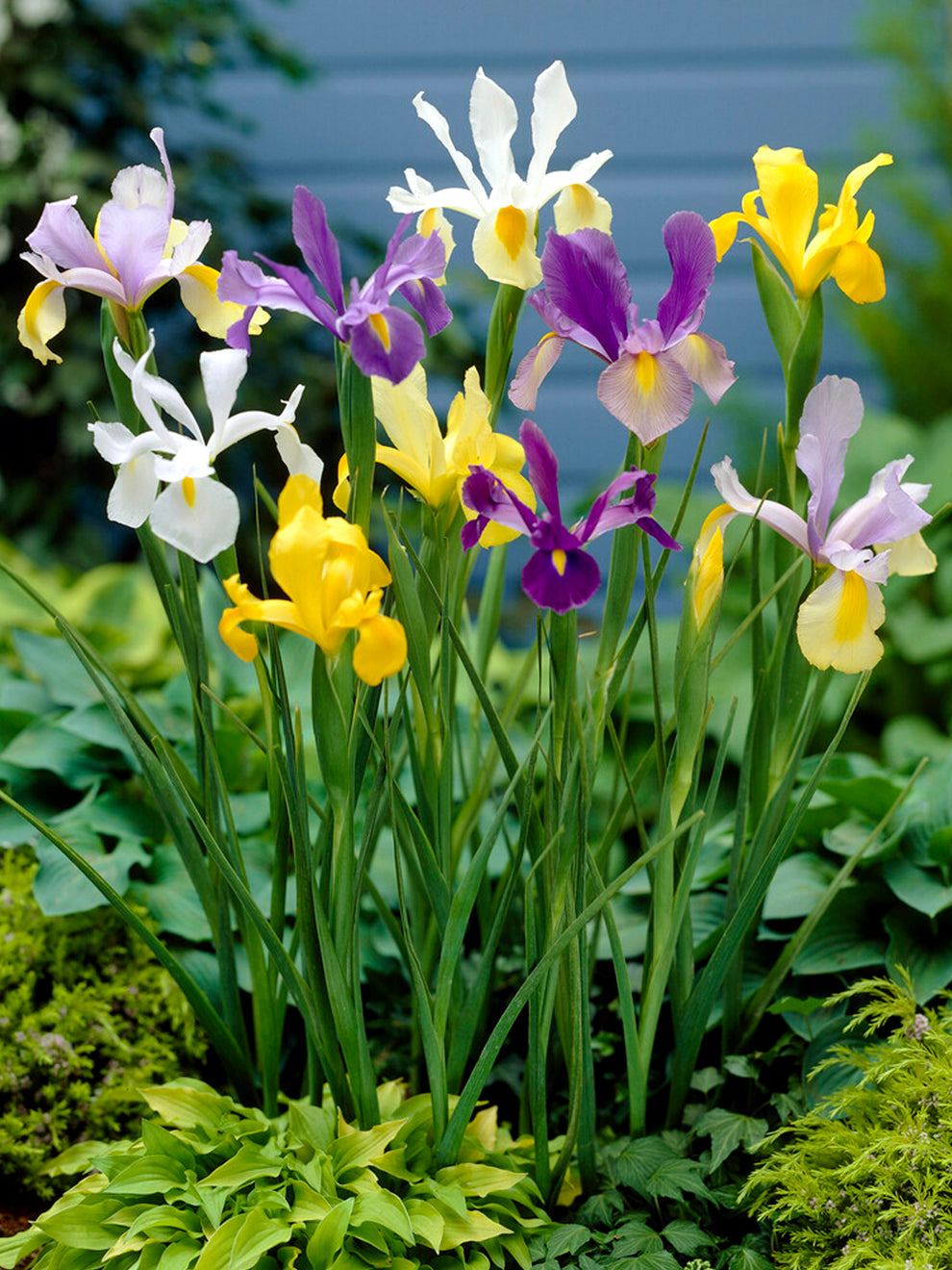The image captures a vibrant garden scene in springtime, focusing on a cluster of freshly bloomed daffodils in a variety of colors. The close-up showcases their healthy green stalks emanating from the ground, surrounded by an array of other green plants in various shades from light to dark. The daffodil stems are notably darker green, while their flower buds exhibit a striking palette of yellows, whites, deep purples, and lavenders, each in different stages of bloom. The background reveals a blurry glimpse of an olive-colored home siding, suggesting the flowers are part of a home garden. Additionally, there are other leaf shapes, including some that resemble oak leaves and a moss-like plant, contributing to the lush, textured greenery around the daffodils. Overall, about 15 flowers are visible, creating a rich and diverse spring tableau.